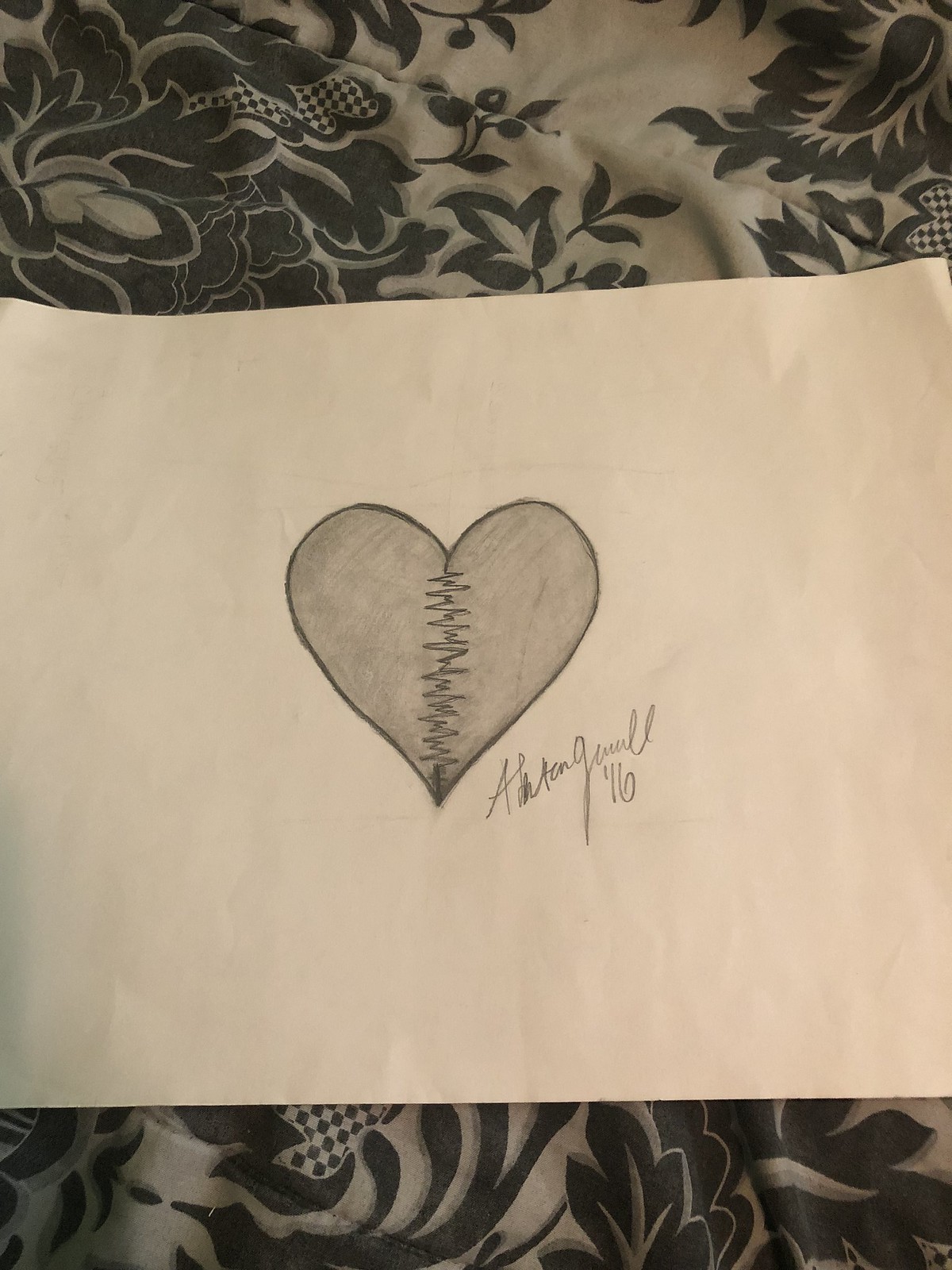The image captures a partially visible horizontal piece of paper positioned on top of a bed, viewed from above. The background features a white comforter adorned with black floral patterns, seen at both the top and bottom edges of the photo. Central to the paper is a detailed pencil drawing of a heart, meticulously stitched along a jagged line as if symbolizing a heart that was once broken and then sewn back together. The heart's outline is heavily reinforced, with the pencil lines repeatedly traced to create a pronounced, bold border. The inner area of the heart is shaded with pencil, adding depth to the drawing. The stitches themselves are depicted with precise pencil lines. To the right of the heart, angled slightly, is a handwritten pencil signature followed by the number "16."